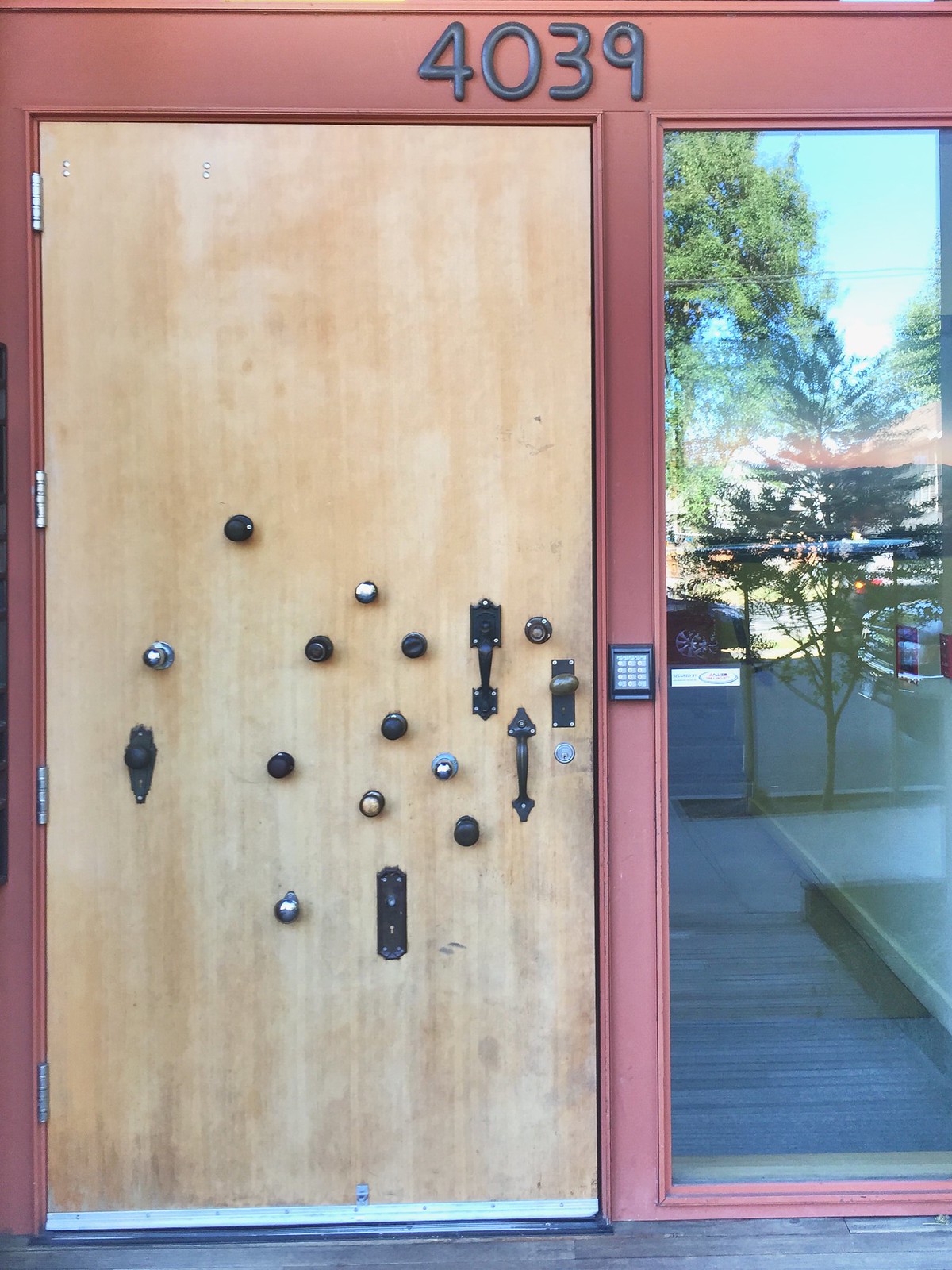The photograph showcases the front of a unique wooden oak-colored door, which features an array of scattered doorknobs and hand pulls mainly concentrated in the middle third of the door. The door is set into a pinkish building facade and is topped by the address number "4039," rendered in black metal type on a red, crimson red wooden surround. Next to the door, there is a tall vertical glass window approximately the same height as the door but not fully visible in the image. Between the door and the window, there is a small gray-buttoned keypad with a black base. The oak door, light brown in color with four hinges, contrasts beautifully with its various doorknobs – more than ten in total – creating a distinctive and unusual appearance. Reflections in the window reveal a glimpse of a blue sky, green trees, and some parked vehicles. The ground below the door is covered with a light brownish-gray wooden floor, adding to the overall visual appeal of this eclectic architectural feature.